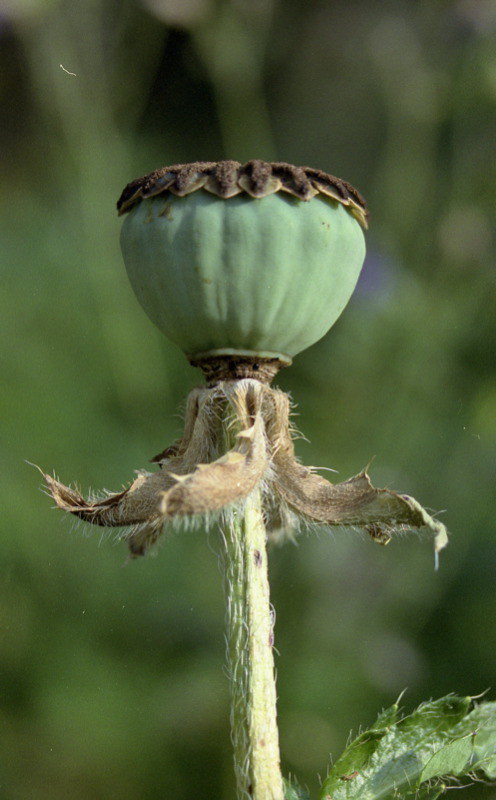The photograph, taken outdoors in portrait orientation, showcases an extremely detailed close-up of a dandelion, notably one of the white puff-headed types often blown on for fun. The dandelion in the image has had its white tufts scattered, either by a gust of wind or someone's breath, leaving only a few scraggly remnants clinging to the lower parts. The focal point is a half-oval bud at the top, featuring a brown, slightly desiccated cap and a green, fluted base. This structure is mounted on a tall, light green stem, adorned with tiny hair-like appendages. In the bottom right of the image, a dark green, pointed leaf with similar white hair-like features can be seen. The background is a blur of greenery, enhancing the subject's vivid detail and emphasizing the photographic representational realism of the shot.